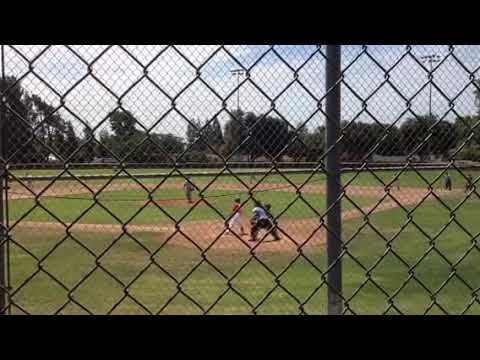The image captures a lively moment at a baseball park, viewed through a chain link fence. It is a clear daytime setting, although the sky is mostly overcast with gray clouds scattered against a blue backdrop. Centered on the photograph, a pitcher is poised to throw a pitch to a batter dressed in a red jersey and white pants. Behind the batter, the catcher and umpire stand in ready positions. The field itself is a vibrant green with a light brown dirt diamond. To the right near first base, both an umpire and a first baseman can be seen, while no players are noticeable in the outfield. Notably, the stands are vacant, and towering light poles stand unlit against the sky. A tree line of green trees frames the background, adding depth to the serene yet dynamic scene. Despite the image’s small size and slight blurriness when zoomed, the details of a Little League game, including black rectangular framing at the top and bottom of the photo, are evident.